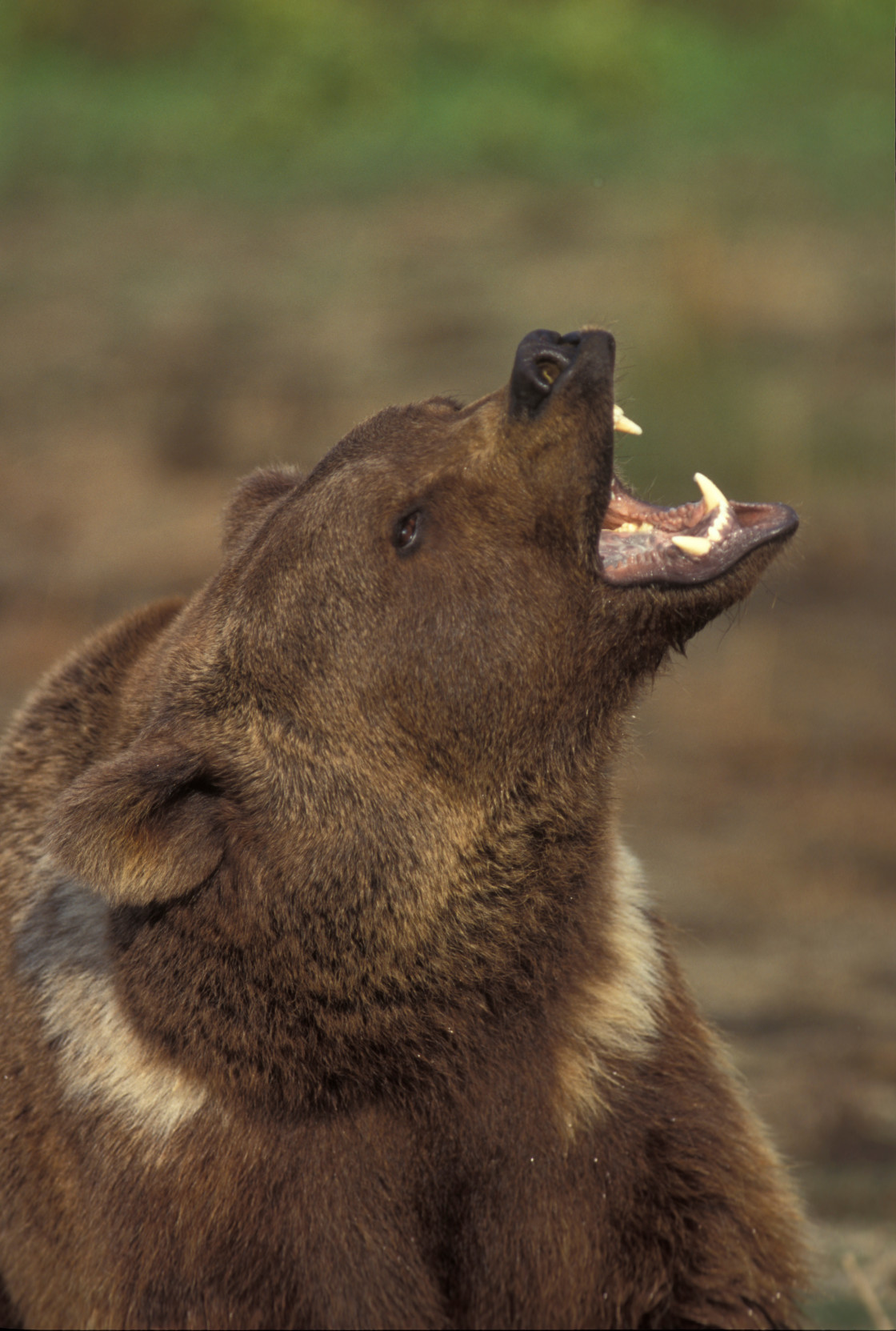This is a highly detailed photo of a brown bear, potentially a grizzly bear, captured in an outdoor, natural setting with a blurred green and brown background. The bear's head is turned up and to the right, its mouth wide open as if roaring or growling, revealing its sharp, off-white teeth with particularly pronounced fangs on both the upper and lower jaws. The bear's fur is predominantly brown with lighter patches, including a fringe of light brown or white around its neck. Its ears have a touch of lighter brown around the tips, contrasting with the darker brown towards the center, and there's notable dark brown shading around its eyes. The bear's expressive profile is highlighted against the blurry, grassy backdrop, showcasing its powerful and striking presence in the wild.